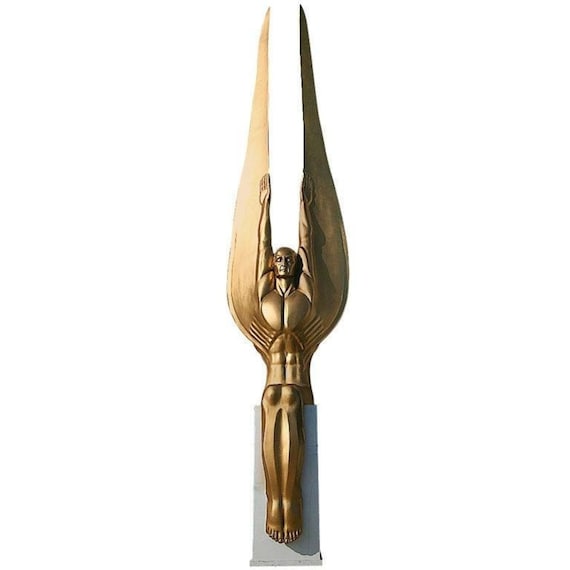The image features a detailed Art Deco angel statue, set against a white background. The statue sits on a vertical, gray, rectangular base that seems to be made from concrete or metal. Perched atop this base is a striking gold statuette. The figure is seated, with bent knees and bare feet pointed downward. The statue's waist is narrow and tapers into a muscular, chiseled torso and a broad chest. The arms are raised straight up beside the ears, with delicate, dainty fingertips pointing skyward. Prominent, smooth gold wings extend from behind the arms, tapering up to sharp points with minor etchings near the base, giving a ribbed appearance. The figure is bald, exuding a sleek, polished finish overall, with distinct, phoenix-like qualities.